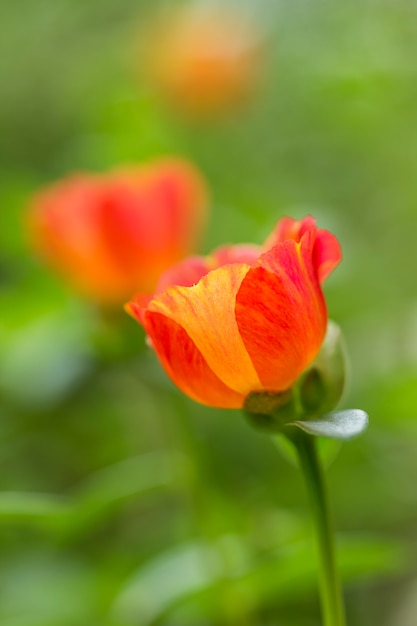This image showcases a stunning close-up of a simple yet elegant orange tulip, with subtle hints of yellow on its cup-shaped petals. The tulip is shown with a green stem and smooth green leaves, centered prominently in the frame. Another tulip can be seen blurred in the background, adding depth to the composition. The background itself is a field of various shades of green, providing a natural, serene setting. The tulip's youthful bloom and vibrant colors evoke a sense of springtime beauty, making it an ideal landing spot for a bumblebee. The photograph is well-composed, capturing the intricate details and textures of the flower's petals and leaves, emphasizing its magnificence against the soft-focused backdrop.